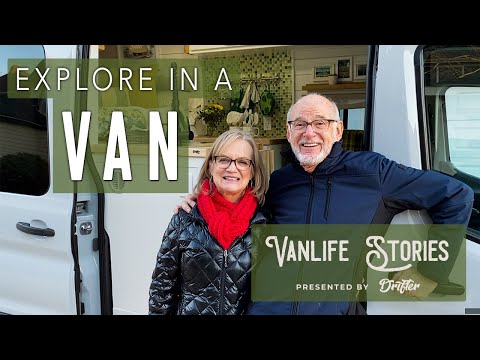The image is a promotional still shot, likely for a YouTube channel called "Van Life Stories presented by Drifter." The photo prominently features an older couple, possibly in their late fifties or early sixties, standing happily in front of a converted Econoline van. The man is balding with a white beard and glasses, and has his hand on the van door handle. The woman, shorter than her husband, is dressed warmly in a black puffer jacket, a red scarf, and also wears glasses. The words "explore in a van" are displayed in white text on a translucent green background in the upper left corner, while "Van Life Stories presented by Drifter" appears on the lower right. Behind the couple, the interior of the van reveals part of a kitchen counter, suggesting it has been transformed into a cozy living space for their life on the road. The image effectively conveys a sense of adventure and companionship, embodying the essence of van life.